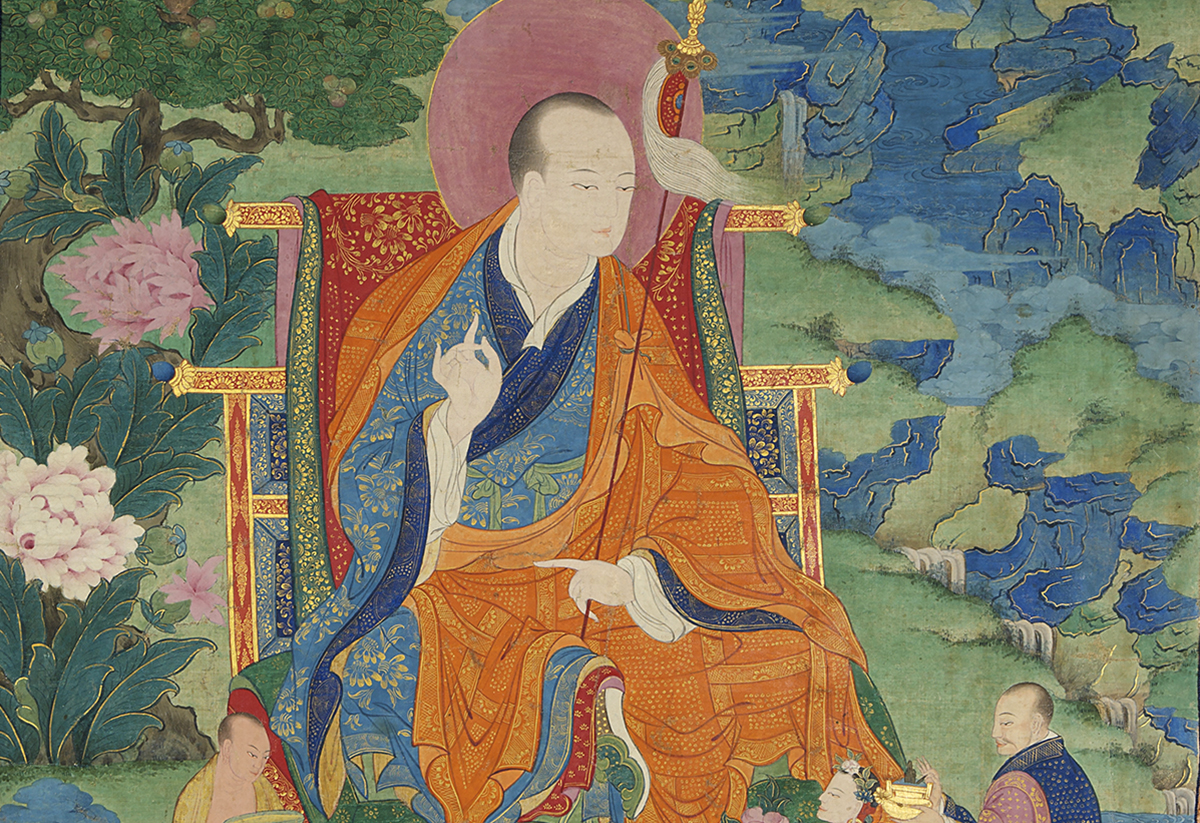The image portrays a detailed and colorful scene, likely an oriental painting or drawing. Central to the picture is a man with dark hair, seated on an elaborate throne featuring dual protrusions at different levels on either side. He dons a multi-colored robe, comprised of a blue undershirt with an orange-goldish outer robe, adorned with gold trims. The throne, rich with detail, has two protrusions at head and shoulder levels, and draped fabric hangs over its back. Behind the man’s head is a purplish circle, perhaps a halo, with a saber-like object visible to the right.

The background is vivid and intricate, filled with pink flowers of various shades, from light pink to darker hues, intermixed with green leaves and designs in blue and green. To the left of the throne, there is a green tree with brown branches and pink flowers, along with some gray rocks. On the ground, there's a blue leaf. To the right, a body of blue water winds among green hills.

At the bottom of the painting, smaller images of three people are visible. To the left of the throne, a man in yellow stands, partially visible from the chest up, looking down. To the right, another figure can be seen shoulder up, looking left. Additionally, there’s a third man dressed in a blue shirt with pink sleeves and yellow details at the bottom right corner of the image. The ornate chair also displays a red, blue, and pink background with gold trim, further enhancing the scene’s rich and lavish aesthetics.